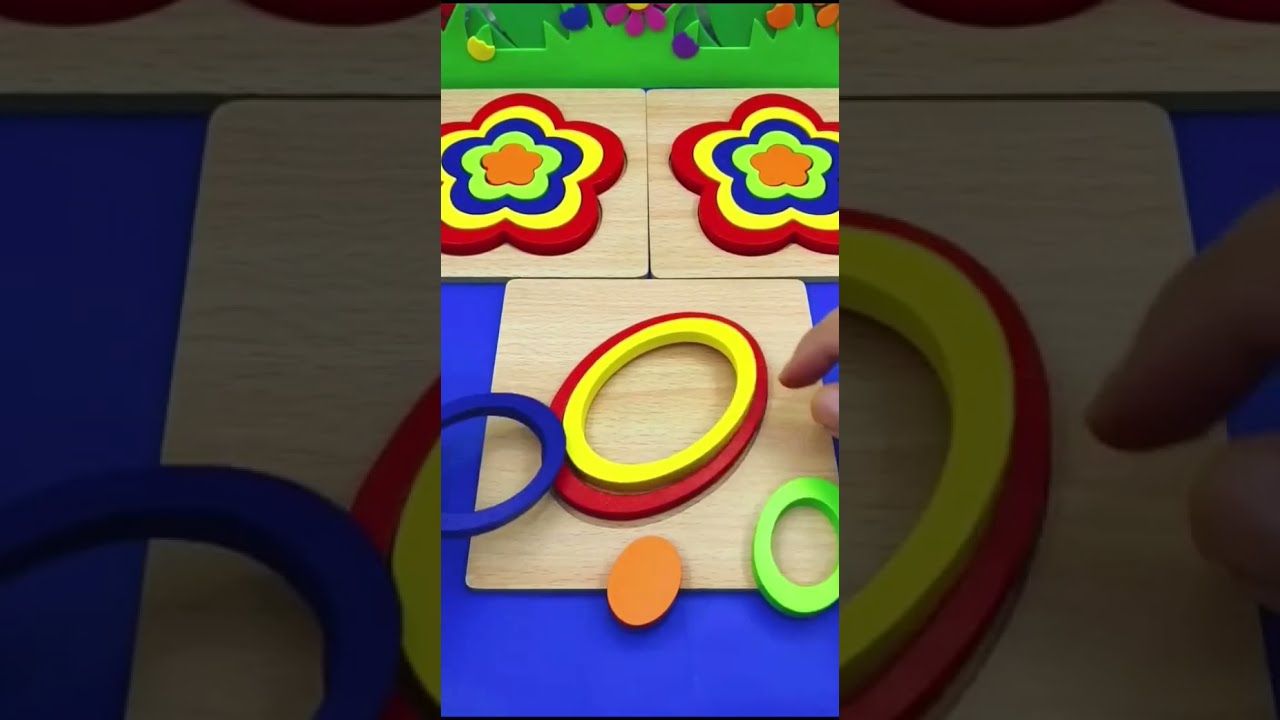The image depicts a vibrant children's puzzle set, arranged on a blue surface. Central to the scene are interlocking oval pieces, each decreasing in size and varying in color from the outermost red, followed by yellow, blue, green, and culminating in a smaller orange piece at the center. Above these ovals are two intricately layered wooden flower puzzles, featuring five petals each. The flowers are composed of multiple interlocking layers of color, starting with the outermost red, followed by yellow, blue, green, and ending in a centrally placed yellow piece. The image captures these toys in a close-up, highlighting their colorful details and assembly complexity, suggestive of a preschool or kindergarten environment.